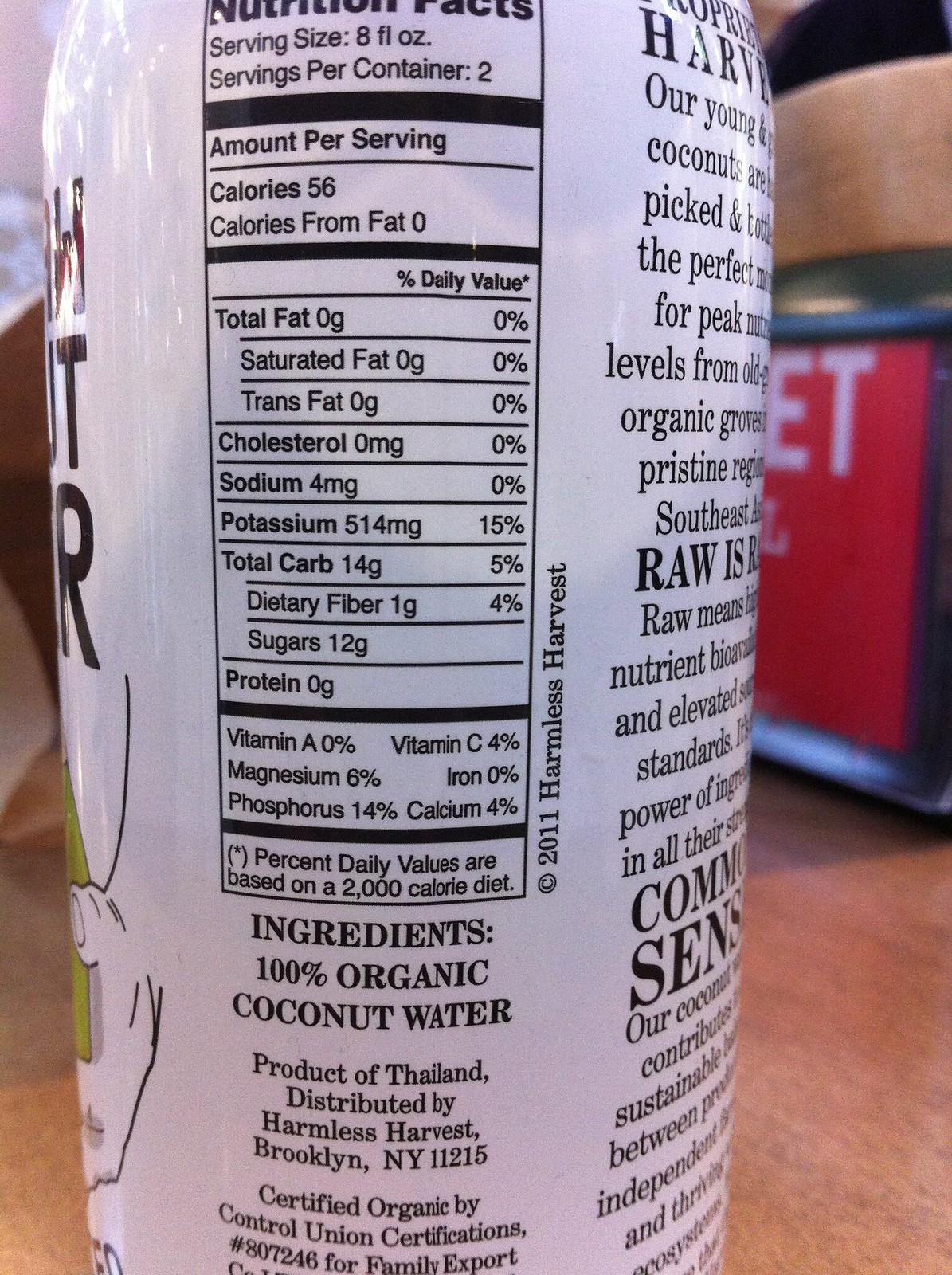This detailed photograph showcases the ingredients section of a white can, prominently displaying the black-lettered "Nutrition Facts" label. The focus is centered on the side of the can where the nutrition information is listed. The serving size of 8 fluid ounces and the fact that there are two servings per container are noted. Additionally, the label reveals that each serving contains 56 calories with zero calories from fat, 514 mg of potassium (15% of the daily value), and 14 grams of total carbohydrates (5% of the daily value).

Beneath the nutritional details, the label lists the ingredients, starting with "100% organic coconut water" and noting that it is a product of Thailand. The distribution information is also provided, stating "Distributed by Harmless Harvest, Brooklyn, New York, 11215" and mentioning certification by Control Union Certifications. The can rests on an orange-brown and tan surface. In the background, towards the right, there is a partial view of a red object with white lettering, including the letters "ET," along with the edge of a black box beside it.